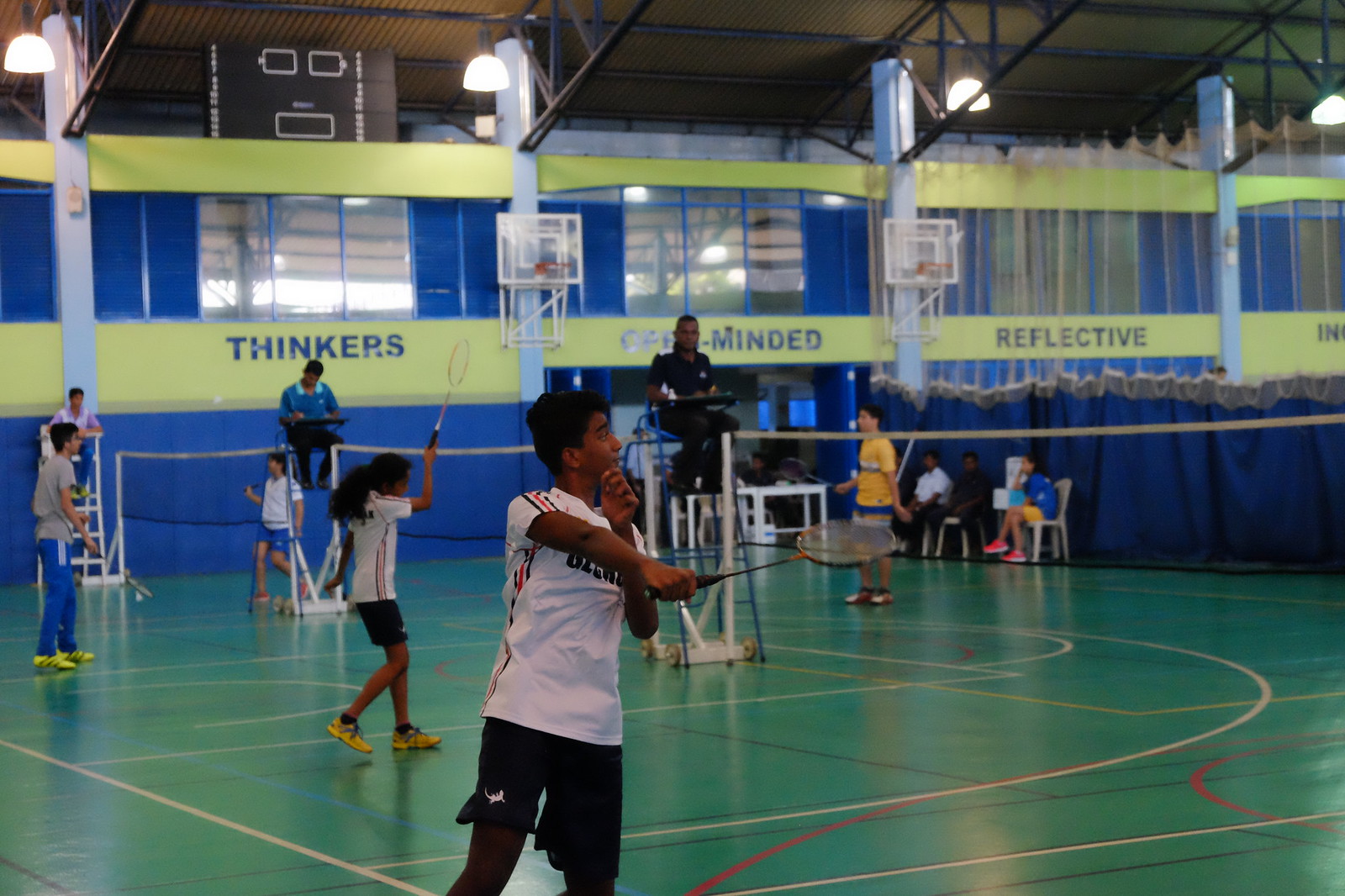This horizontally aligned rectangular picture captures an indoor badminton tournament in a brightly lit gymnasium. The green floor is crisscrossed with a network of yellow, red, and white curved lines. Three separate badminton courts are set up with nets stretching across the middle of the picture. Players, who appear to be teenagers from various racial backgrounds including white and Asian, are actively engaged in their matches. On the left side of the image, two teammates, both donning white shirts with black stripes down the sides and black shorts, are visible. Their opponents, wearing yellow shirts, can be seen on the other side of the nets. Each court has a referee perched on tall seats at the ends of the nets, overseeing the games.

In the background, the gym's walls feature a colorful display: the lower section is blue, followed by a yellow stripe with large printed words such as "thinkers," "open-minded," and "reflective." Above this middle yellow section, another blue area is punctuated by windows leading to an upstairs section, and there is an additional yellow strip above. A black scoreboard is situated at the far end of the gym, and bright lights hang from the rafters, illuminating the entire scene. The combination of the dynamic sports action and the vibrant background creates an engaging and lively atmosphere in the photograph.